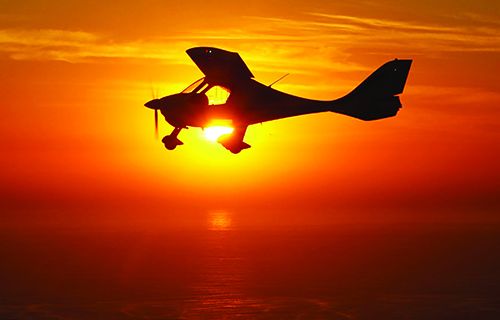This vivid, color photograph captures a mesmerizing scene at sunset, dominated by brilliant shades of reddish-orange. Against this vibrant backdrop, a smaller aircraft, resembling either a small civilian plane or an experimental craft, is prominently silhouetted in profile, appearing almost like a dark silhouette. The sky is adorned with a glowing yellow sun radiating intense light, which diffuses outward into an expanse of warm hues, transitioning from golden yellow to deeper reds. Clouds are sparingly scattered at the top of the frame. Below the aircraft, there appears to be a body of water reflecting the sky's fiery colors, enhancing the image's dramatic ambiance. Despite the sun's intense glow making the details of the aircraft hard to discern, the overall composition, with its dynamic interplay of light and shadow, creates a stunning visual where the aircraft stands as the central focal point amid a picturesque sunset, seemingly enhanced by a filter that intensifies the scene's orange tones.